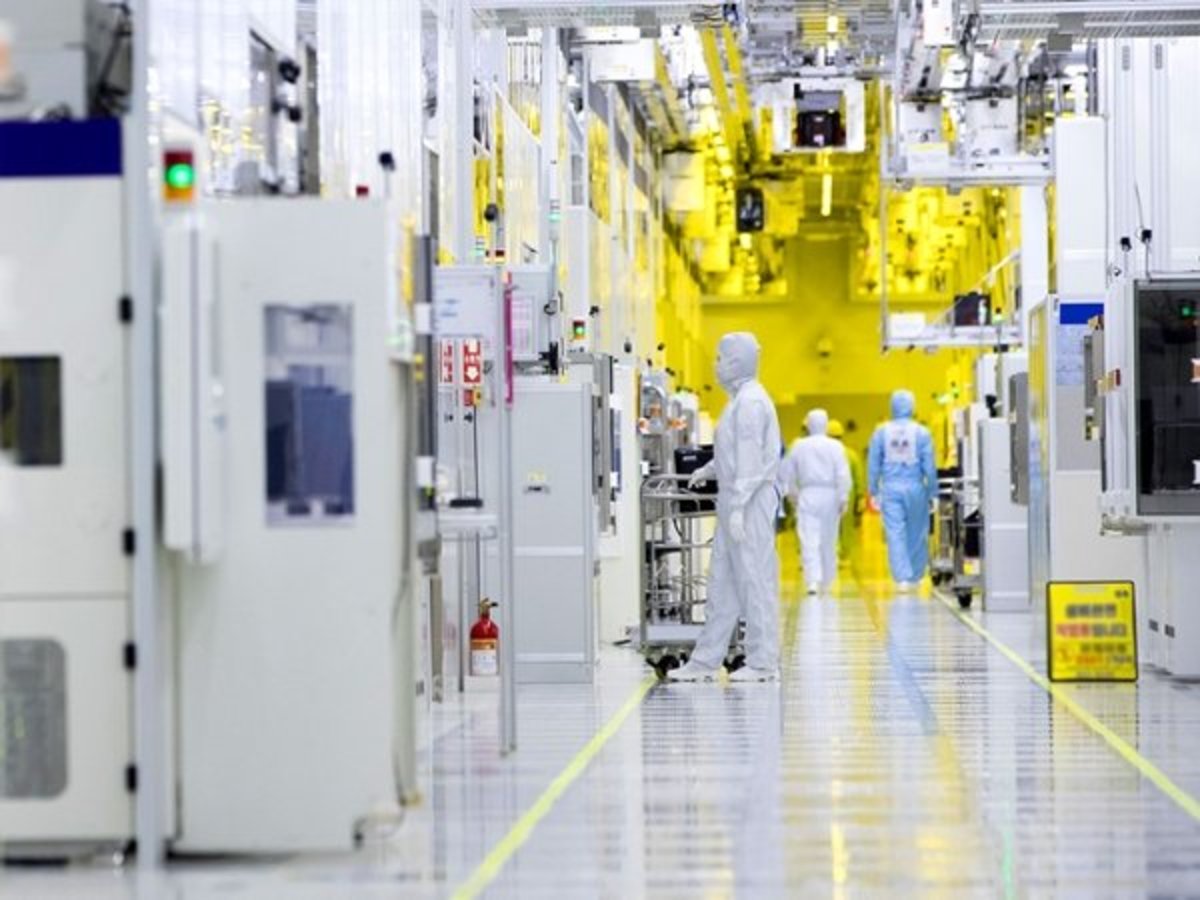The image depicts the interior of a high-tech, possibly biohazardous or clean room laboratory, potentially involved in semiconductor manufacturing or pharmaceutical production, situated in an Asian facility, suggested by the presence of Asian script on a sign. The environment exudes a sterile and highly controlled atmosphere, characterized by bright white, reflective flooring and complex machinery lined along both sides of the spacious hallway. The rear wall and portions of the ceiling are illuminated with fluorescent yellow lighting, enhancing the clinical ambiance. On the left, a fire extinguisher is visible, and on the right, there's a cautionary floor sign with black and red writing. Central to the scene is a man clad entirely in white protective gear—white from head to toe including his sneakers, gloves, and mask—standing and holding a cart with his right hand. Two other individuals, one dressed in white and the other in blue hazmat suits, are seen walking away from the camera, emphasizing the stringent safety measures adopted within this sterile workspace. The overall setting is immaculate and orderly, ensuring strict adherence to cleanliness and contamination control protocols.